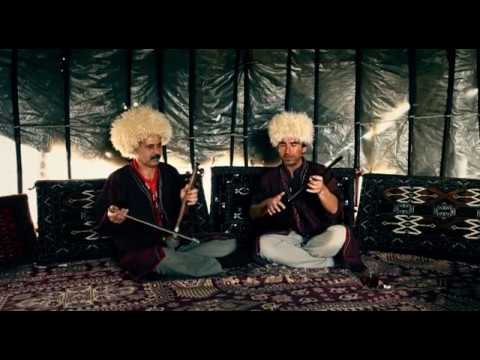In this blurry photograph, two men are captured sitting cross-legged on a richly designed Persian or Turkish rug. They are seated on a large, four-section seat, both occupying the middle sections which have intricate black and white designs. Each man wears a large, fuzzy, cream-colored hat and a dark (possibly black), almost cloak-like jacket – the one on the left featuring a red shirt underneath, and the one on the right lighter-colored pants. In their hands, they hold metal objects resembling the barrel part of a gun or the handle part of an umbrella; the man on the left holds two crossed together, while the man on the right holds just one and seems to be closing his eyes. They are seemingly playing a stringed instrument. A designed Persian rug lies beneath them, and the background includes reflective, silvery material giving the appearance of aluminum foil or some form of insulation, which fades from a black ceiling to gray. Light subtly illuminates the scene from the left-hand side. Pillows with tribal designs are placed behind them, contributing to the cozy and artistic setting. The man on the left sports a mustache, enhancing the distinctiveness between the two.